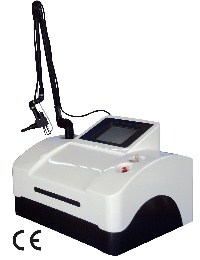The image depicts an electronic measuring device with a predominantly off-white, box-like body and a black base. The rounded top features a small rectangular LED screen with a black frame. To the side of the screen, there's a prominent red button with a switch situated above it. The front of the device houses a black slot, hinting at an inlet or outlet function. Extending from the opposite side of the button is a large, crane-like arm, which can be adjusted and bent, ending in a pointed tool. A wire connects the crane arm to the LED screen, suggesting a functional relationship for measurement purposes. The bottom left corner of the device is marked with the letters "CE," indicating its certification.